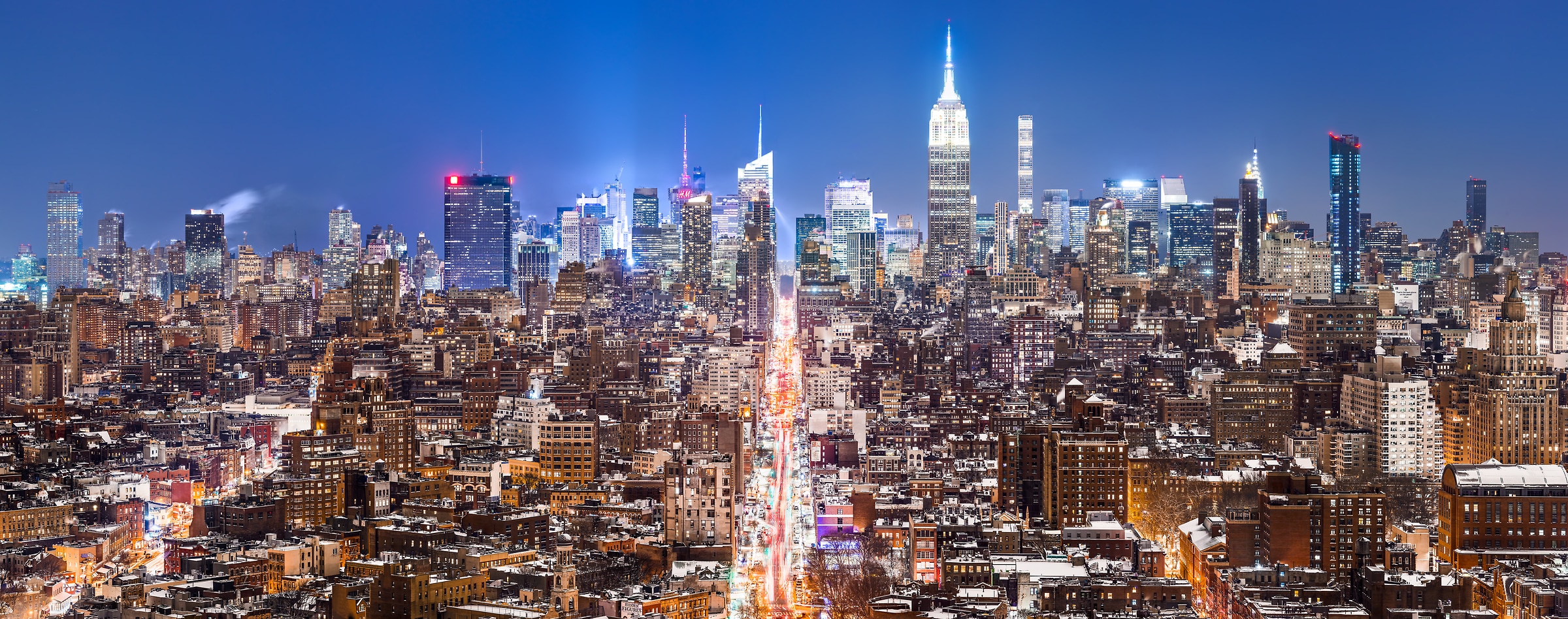This image captures a bustling city skyline, likely of New York City, taken from a bird's eye view or perhaps from a helicopter at night. The scene is dominated by countless buildings of varying heights, which increase towards the background, culminating in towering skyscrapers. Among these, some show recognizable features, possibly including the Empire State Building and the Freedom Tower, although identification is uncertain. The sky is a dark blue, illuminated by the extensive city lights that contribute to significant light pollution, casting a glow that brightens the backdrop. The city's vibrancy is further evidenced by a busy street running through the center, with fast-moving cars that create streaks of gold from their headlights. White lights atop several buildings punctuate the scene, some adorned with red lights at their peaks. Overall, the predominant colors are the golden hues of the car lights and the white lights from the illuminated buildings, giving the city a lively and dynamic nighttime appearance.